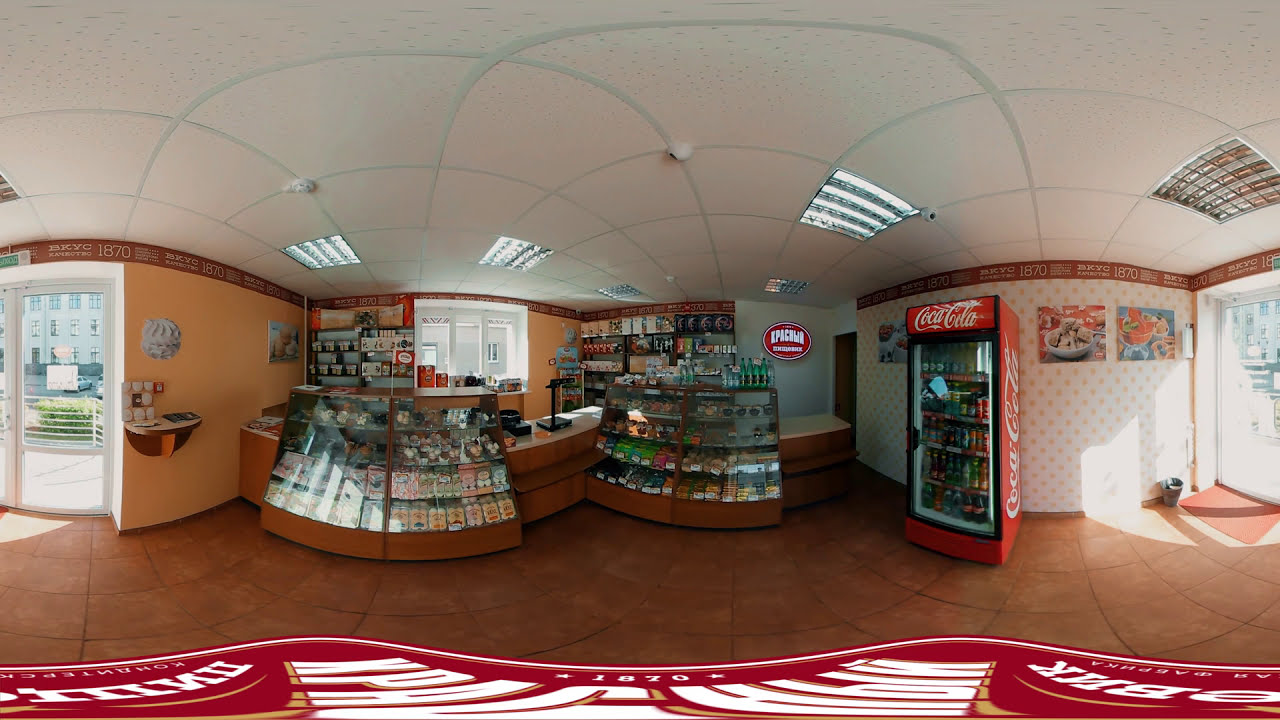The image portrays the interior of a bakery-like convenience store with varied elements. Dominating the left side is a glass display case showcasing multiple pastries, such as cupcakes and donuts, resting on a wooden foundation. The store has a white background wall adorned with orange and peach-colored patterned wallpaper. To the right side of the image stands a red Coca-Cola vending machine filled with bottled sodas. Scattered throughout the store are multiple shelves stocked with various candies and other items, each tagged with white price labels. A cashier counter equipped with a register and possibly a phone is situated centrally, and an additional product stand is visible in the corner. The floor features brown tiles, and closer to the front, there is a carpet with some lettering. There is also a door leading outside to a neighboring building with multiple windows, and several banners with text hang on the walls, adding even more detail to the environment. The ceiling features a sign, whose content is indiscernible, further emphasizing the store's identity.